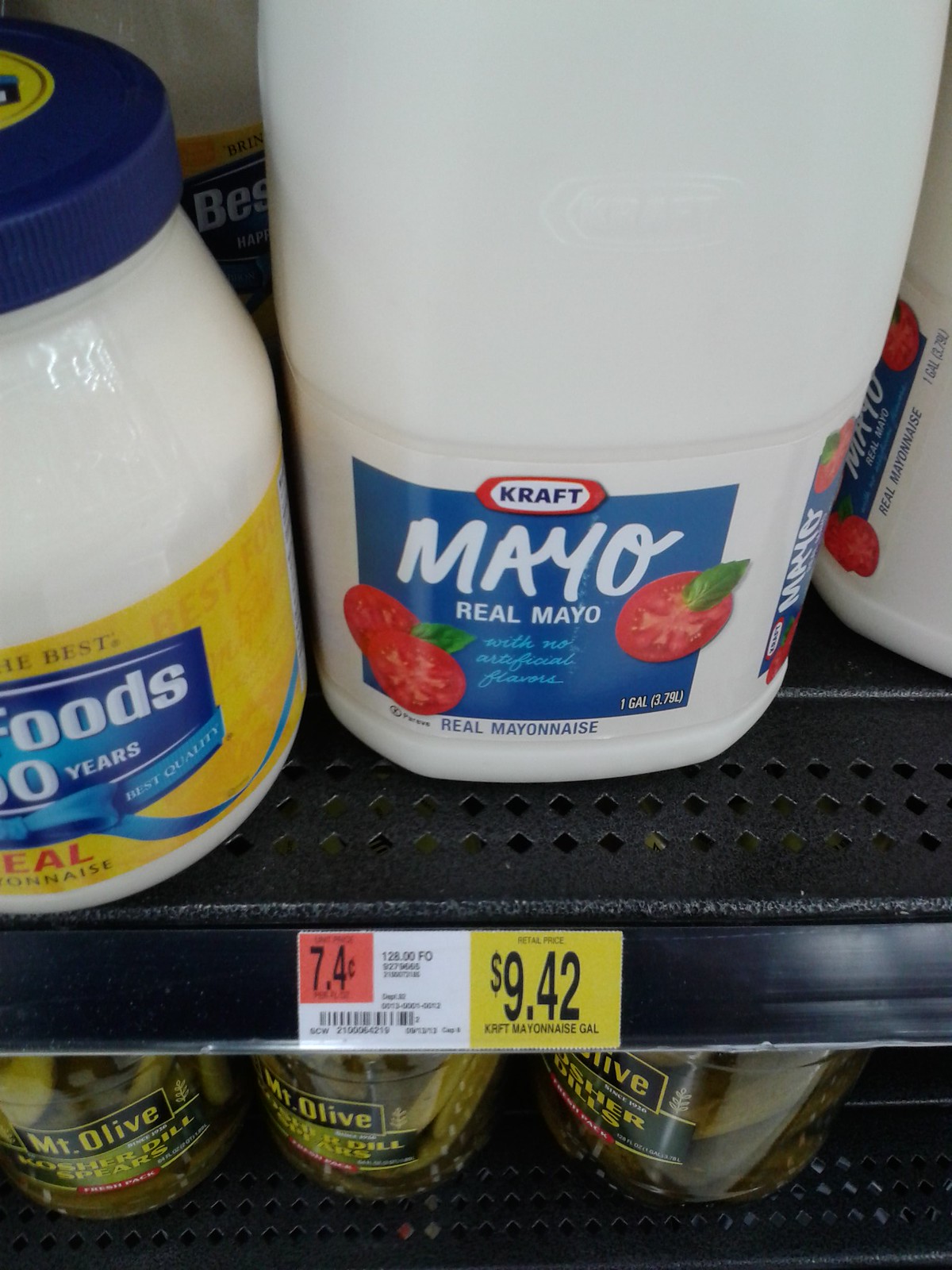The image shows a grocery store shelf, likely from Walmart, displaying a selection of mayonnaise and pickles. The main focus is a large, one-gallon jug of Kraft Real Mayo in a white container with a blue label. The label, which says "Real Mayo" in white text, also features images of sliced red tomatoes, one on the right and two on the left, each adorned with basil leaves. Priced at $9.42, this giant mayo jug stands prominently on the shelf. To the left of it is a normal-sized jar of mayonnaise, possibly Hellman's or Best Foods, and to the right, the edge of another similar-looking mayo container is visible. Below on a shelf with black, diamond-shaped holes are three jars of Mount Olive Kosher dill spears pickles. The shelf tag clearly indicates the price, displaying a half-yellow, half-white label with additional small print and a red square that says "7.4 cents." The overall image emphasizes the size and brand of the mayonnaise, along with the organized arrangement of products on the metal shelving.